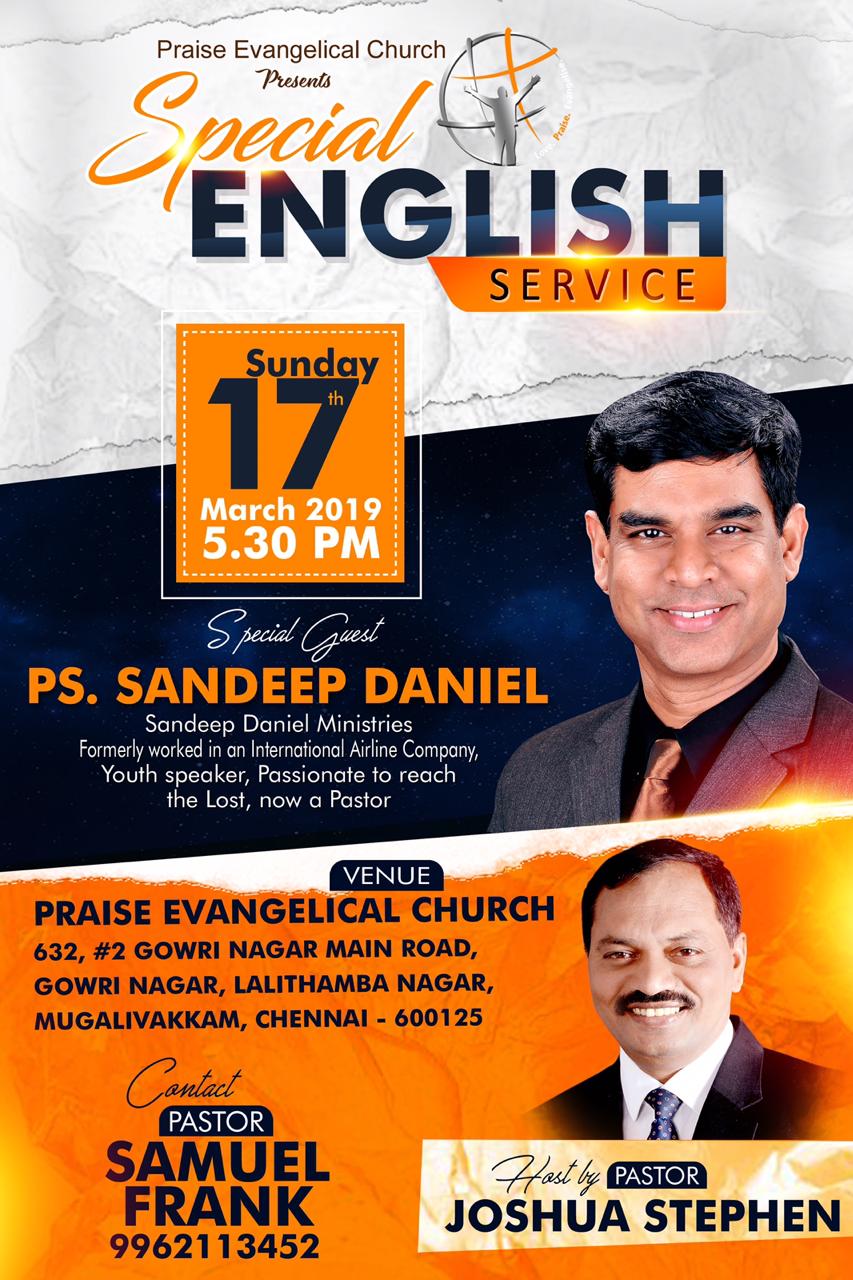The promotional poster features an advertisement for a special English service hosted by Praise Evangelical Church, scheduled for Sunday, 17th March 2019 at 5:30 p.m. The event will have special guest PS Sandeep Daniel from Sandeep Daniel Ministries, who is described as a former international airline company employee, a youth speaker passionate about reaching the lost, and now a pastor. The top portion of the flyer includes a headshot of PS Sandeep Daniel, an Indian male in his 30s or 40s, smiling, dressed in a dark gray suit, a black dress shirt, and a shining bronze tie. Below his image, there is a profile picture of another Indian male, seemingly older, with short black hair and a mustache, also dressed formally in a black suit, white dress shirt, and dark blue tie, smiling directly at the camera. The venue for the event is listed as Praise Evangelical Church, located at 632, Number 2, Gowri Nagar Main Road, Gowri Nagar, Lalit Habamba Nagar, Mugalivakkam, Chennai, 600125. The flyer also provides contact information for Pastor Samuel Frank (9962113452) and mentions that the event is hosted by Pastor Joshua Stephen. The poster is visually segmented with three background stripes in white, dark blue, and orange, and the color palette includes gray, black, dark blue, white, and orange.